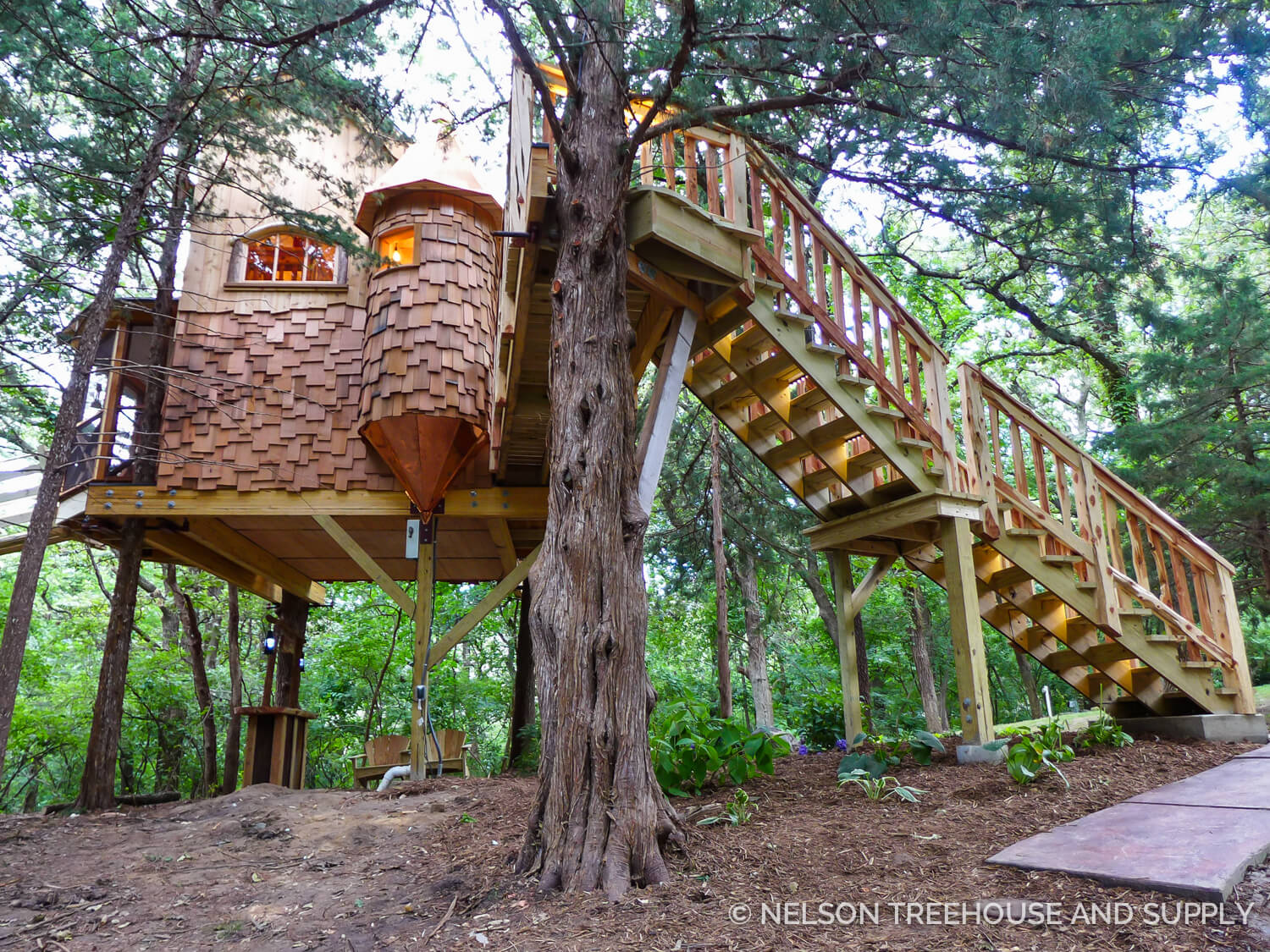The photograph showcases a strikingly beautiful and sophisticated treehouse set against a background of tall, ancient, evergreen trees with dense, green foliage. Occupying the central and right portions of the image, a large tree supports the treehouse, which is raised approximately two meters off the ground, accessed by a staggered wooden staircase. The structure, clearly crafted by skilled carpenters, features intricate details such as individual bark shingles, highlighting its professional build. The treehouse includes two illuminated glass windows, emanating a warm, yellow light that adds a sense of coziness to the scene. The bright sky and natural daylight emphasize the clarity and color of the photograph, which also includes the text "Nelson Treehouse and Supply" with a copyright symbol in the bottom right corner, indicating the photo was taken by the company as a display of their craftsmanship.